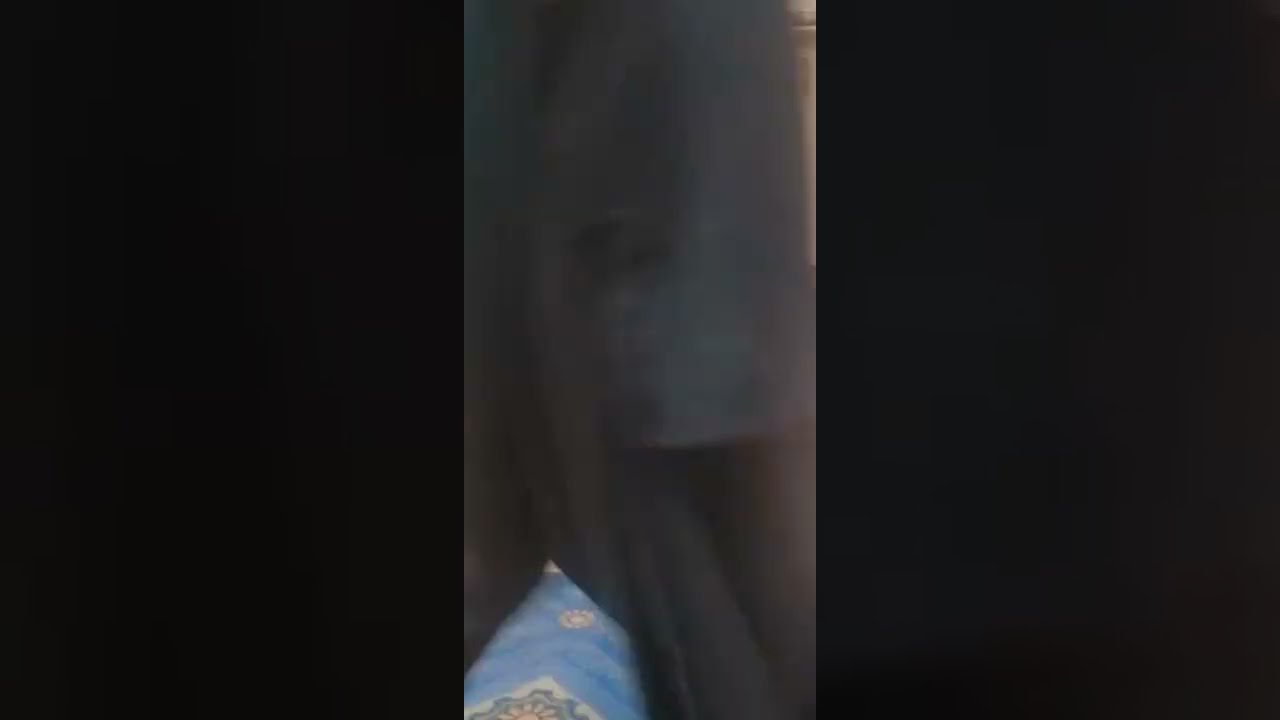The image is framed by large black boxes on the left and right, making the actual photo a vertical strip that is thinner than the black borders. The photo itself is very low quality and blurry, adding to the difficulty in discerning its contents. At the bottom left corner, there appears to be a blue bag, possibly a bag of sugar, with a bit of white at the front but no visible text. Above this blue bag, there is a gray, robe-like garment dominating the center, which has a swirly, almost geometric pattern with a beige disc in the center resembling a bathtub drain. In the same corner, partially visible, is what seems to be a pillow with a floral design. The predominant colors in the image are shades of gray and darker tones, contributing to its overall obscured and indeterminate appearance.